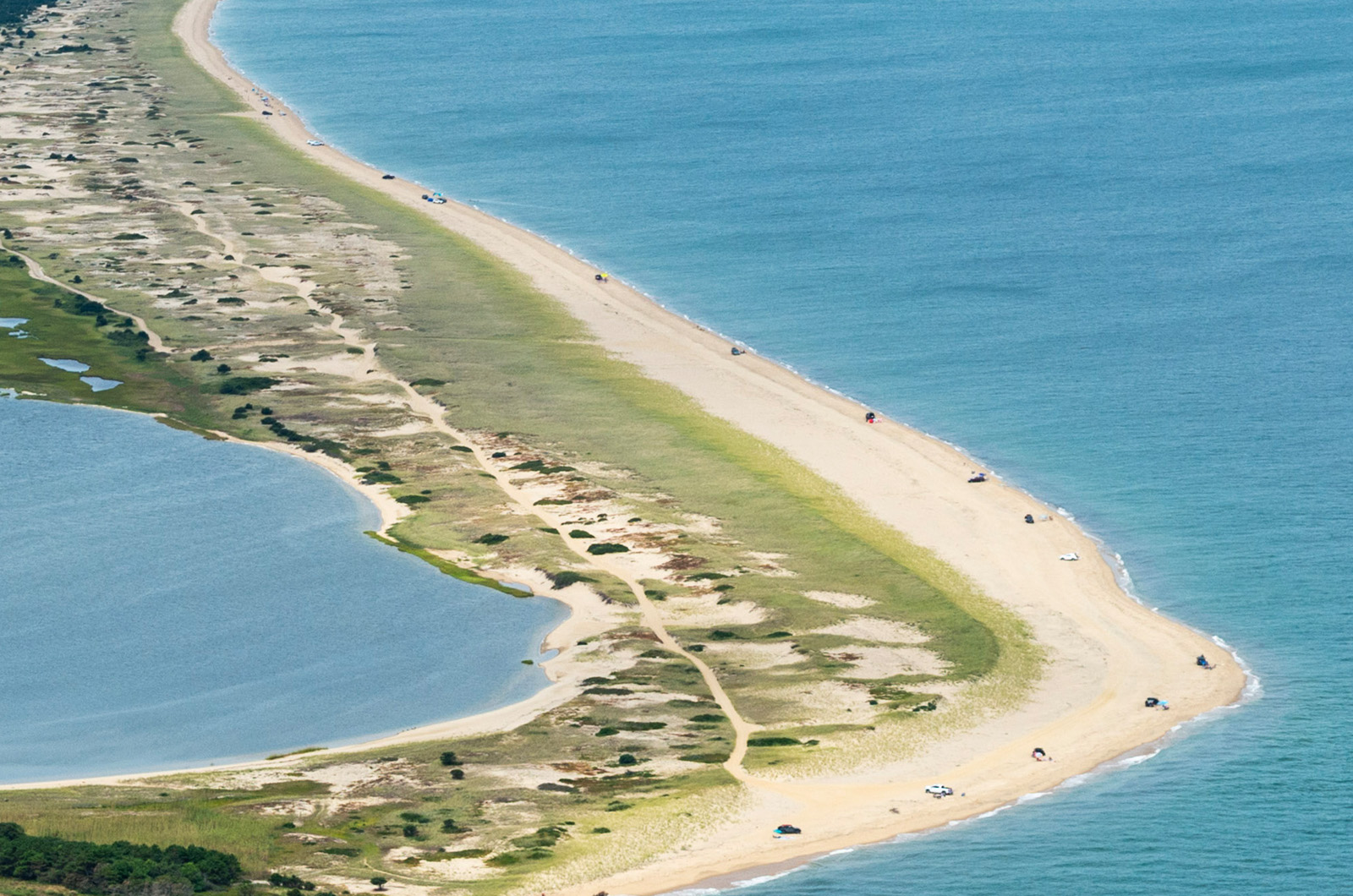This aerial image captures a vibrant, curved landmass jutting out from the upper left to the lower right, then hooking back to the lower left. The strip of land boasts lush green areas interspersed with sandy trails, transitioning into a long, light brown shoreline. On this expansive beach, evenly spaced cars and beachgoers with their belongings dot the sand. Tall trees cluster at the lower left, adding to the greenery. Surrounding this landform are two striking blue waterways, one on each side, creating a picturesque divide between the lush island and the vast body of water. The sea is a rich medium blue, filled with ripples, while the crystal-clear beach waters enhance the natural beauty of this sunny outdoor scene. The sky is not visible in the photo, focusing the viewer's attention on the contrasting colors and textures of the landscape and water.